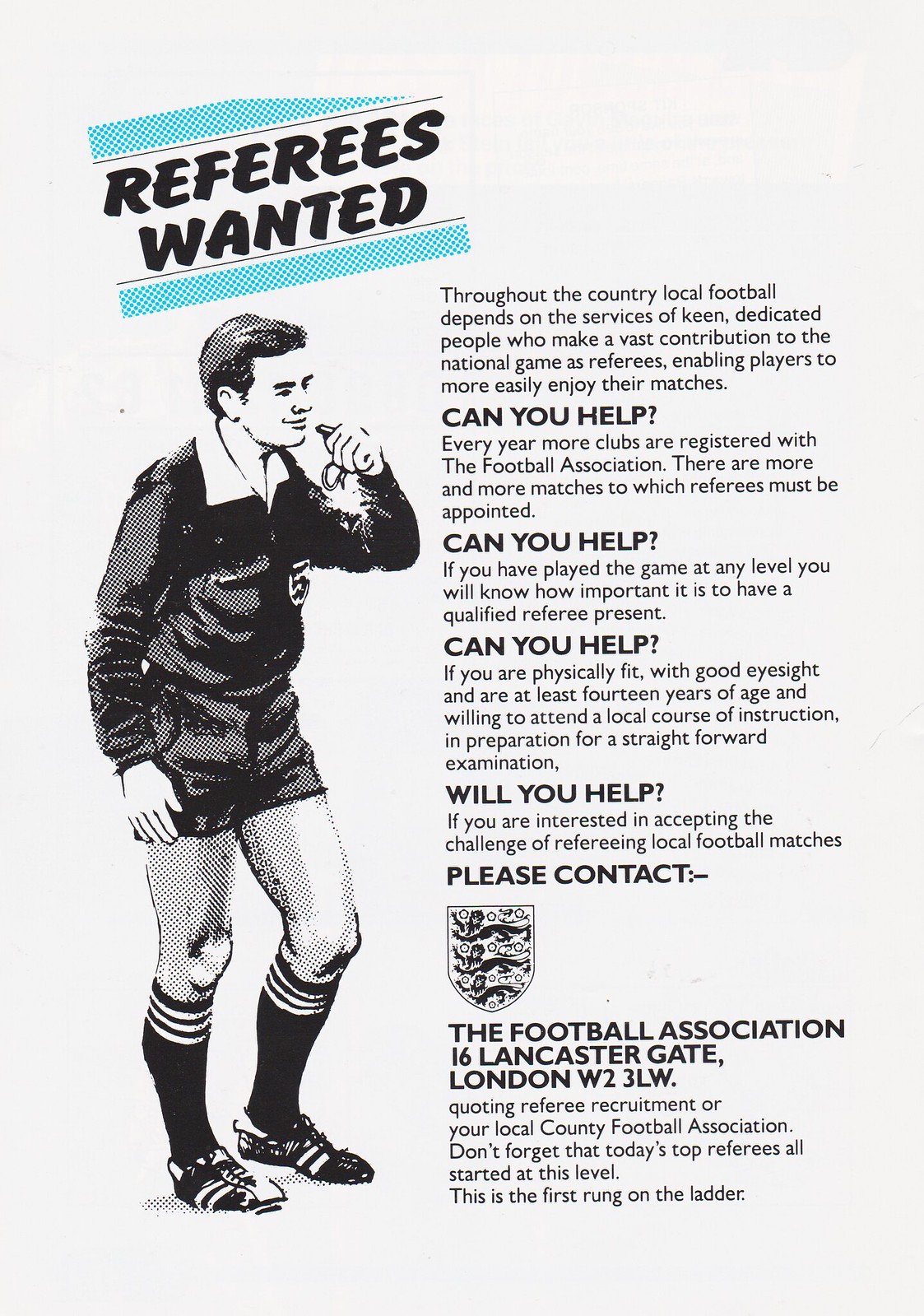This vintage recruitment poster for referees, set against a white background, prominently features a bold, black "Referees Wanted" headline at the top-left, flanked by blue bars above and below the text. The central illustration, a pencil-drawn figure of a referee, shows him clad in dark attire – a long-sleeved top, shorts, thigh-high socks with white stripes, and dark running shoes. He has short, dark hair and is raising a whistle to his lips with his left hand. To the right of the drawing, a detailed message articulates the essential role of dedicated referees in local football, encouraging individuals to contribute to the national game. The text emphasizes several times with phrases like "Can you help?" and "Will you help?" urging potential referees to get involved. At the bottom, contact information is provided, notably listing "The Football Association, 16 Lancaster Gate, London, W23LW," indicating a pre-digital era contact method.